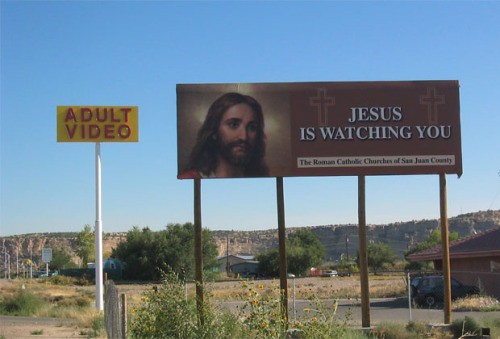The image depicts a desert-like landscape featuring a prominent brown billboard supported by four wooden posts that blend with the parched backdrop. The billboard prominently displays a picture of Jesus on the left side, flanked by two crosses. The right side of the billboard reads in white letters, "Jesus is watching you." Beneath, it identifies the Roman Catholic Church of San Jose County. Adjacent to this, on a tall white pole, there's a yellow rectangular sign with red lettering that reads "adult video." The landscape showcases a mix of low-lying trees, dead grass, and several houses, with a mountain range and clear blue sky in the background, highlighting the stark contrast between the religious message and the adult video advertisement.